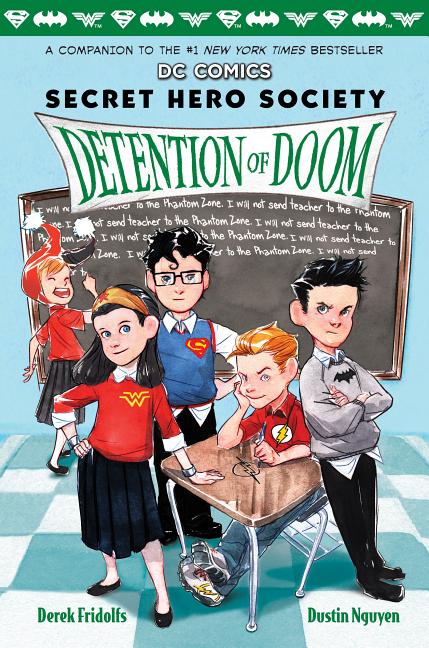This digitally-created image features a group of children in a classroom, likely the cover of a companion book to the number one New York Times bestseller, "DC Comics Secret Hero Society: Detention of Doom." The top of the image has a strip of green with repeating logos of Superman, Batman, and possibly Wonder Woman. The text in a unique font reads "DETENTION OF DOOM" on a white, stretched-out rectangle.

The classroom scene includes five children and a teacher at a chalkboard. A boy in a blue shirt with the Superman 'S' logo is front and center, his black hair contrasting with his white collar. A girl with a red Wonder Woman shirt, black skirt, cufflinks, and a bandana stands confidently. Another child sports a gray Batman logo shirt, and a fourth, sitting at a desk, wears a red Flash logo shirt. A fifth character, a male with orange hair, wears glasses. The teacher appears to be writing on the black chalkboard.

The colors in the image are varied, including green, white, light blue, black, gray, red, yellow, and orange, enhancing its vibrant cartoon style. The names "Derek Fridolfs" and "Dustin Nguyen" are noted at the bottom, indicating the creators. This image captures a lively moment indoors with a clear comic book aesthetic.